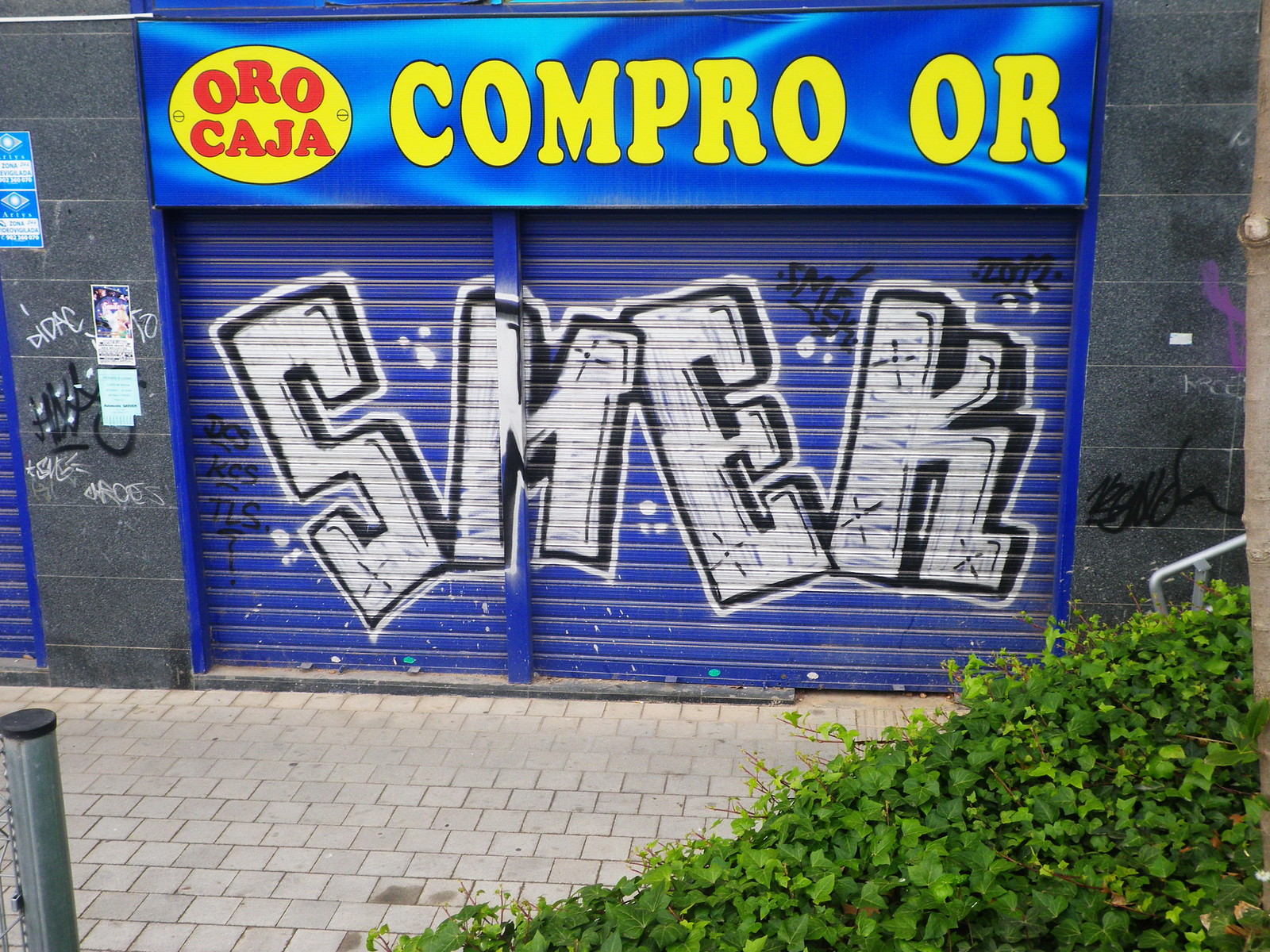The photograph captures an outdoor scene featuring a shuttered storefront with a blue roll-up door covered in graffiti. Centered above the door is a blue sign, divided into two sections: a yellow oval on the left with the bold red text "ORO CAJA," and on the right, in large yellow letters, it reads "COMPRO OR." Prominent black and white graffiti spells out "SMEK" in large, 3D-style letters with small dots around them. The storefront is framed by a smooth, slate gray wall, which also sports additional graffiti. The ground in front of the store is a faded, gray brick sidewalk, once red, and includes a gray pole and a metal handrail on the right. There's a bushy green plant in the bottom right corner, hinting at some greenery amidst the urban setting. Adjacent to this storefront, there's another blue door visible to the left, suggesting the presence of multiple storefronts in the vicinity.